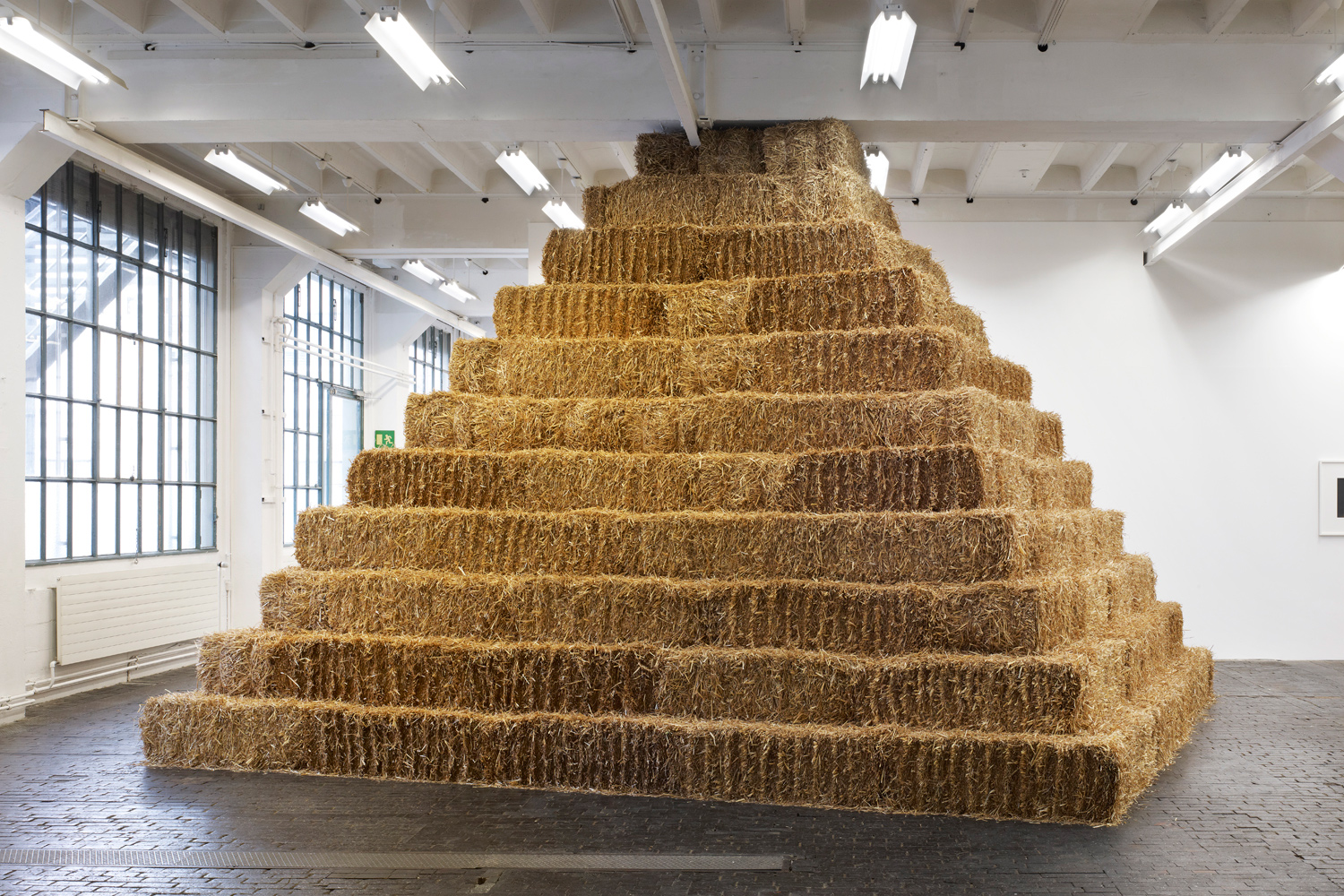This photograph captures an intriguing scene of a large pyramid structure meticulously crafted from hay bales, stacked in eleven distinct layers reaching up to the ceiling. Set within a room with very bright white walls and a gray brick or dark wood floor, the space resembles a commercial or industrial setting, possibly a museum or a warehouse. The room is well-lit by big fluorescent lights hanging from the white ceiling, enhancing the golden yellow hue of the hay. On the left side of the room, there are large industrial windows with bars and frames painted black, contributing to an austere, prison-like ambience. A green sign is faintly visible behind the hay on the wall, though its text is indiscernible. The geometric, staircase-like arrangement of the hay bales evokes the form of an Aztec pyramid, presenting an abstract, sculptural art piece amidst the stark surroundings.